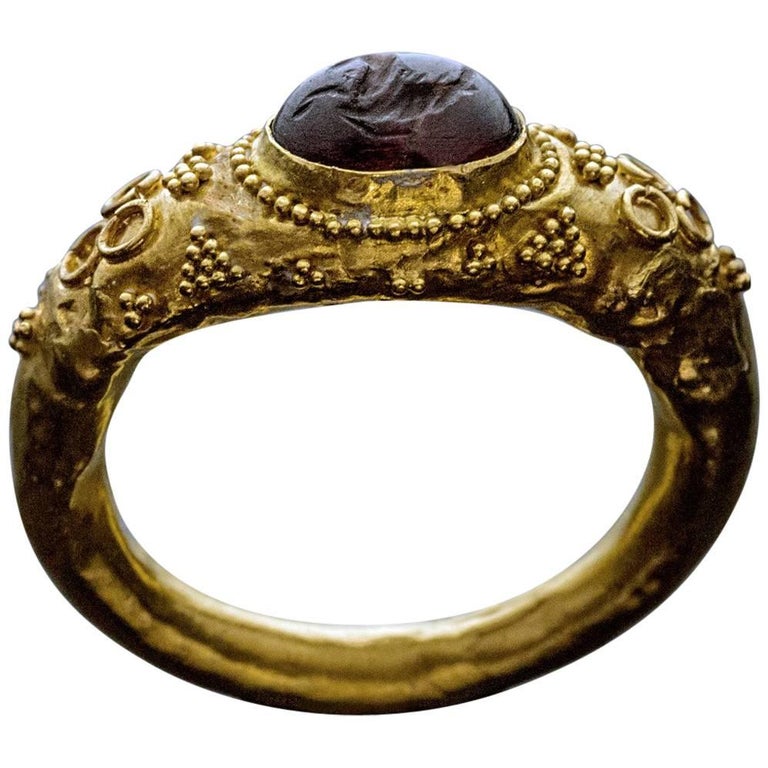The image showcases an intricate ring with a striking goldish hue, floating against a pristine white background. Dominating the ring is a substantial, oval-shaped black stone centrally set atop a thick, somewhat rough band. This inky black stone, exhibiting engravings and polished to a subtle sheen, appears slightly gouged in the middle, adding character and depth. Surrounding the stone, the top of the band is adorned with clusters of small, gold beads arranged in triangular shapes, creating a rich decorative effect.

The band's design is minimalistic along the sides and bottom, distinguished by its flat, uniform structure, although the gold appears slightly wavy, indicating potential age and artisanal craftsmanship. The ring seems to possess a historical, artifact-like quality, reminiscent of pieces found in museums, hinting at its antiquity and the hand-forged nature of its creation. The angle of the image reveals both the top detailing and partially the ring's interior, primarily on the right side, offering a comprehensive view of this unique piece. The simplicity of the white background ensures that all attention is on the ring and its elaborate upper design.